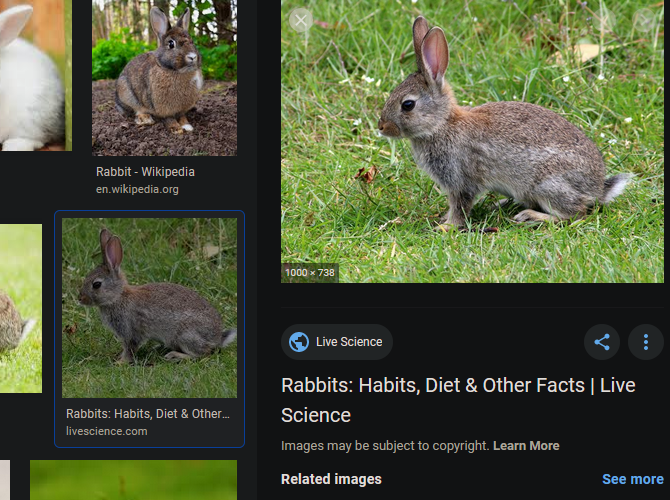The image features a collage of various depictions of rabbits, accompanied by descriptive text and web links. In the upper left corner, a white rabbit is partially visible, showing only its back and one ear. To its right, a brown rabbit is prominently displayed, characterized by a distinctive white spot on its chest, a white nose, and one white paw, while the rest of its body remains brown. Beneath these images, there is a reference to "Rabbit Wikipedia" with a link to en.wikipedia.org.

Further down, another frame displays a gray rabbit with a white tail, facing left and standing in a grassy area. This frame is outlined in blue and includes a caption beneath the rabbit reading "Rabbits, habits, diets, and others..." with a link to lifescience.com. To the right of this is a larger version of the same gray rabbit image, with the dimensions 1000 by 738 noted on the lower left side. Beneath this larger picture, text reads "LifeScience," followed by "Rabbits, habits, diets, and other facts at LifeScience."